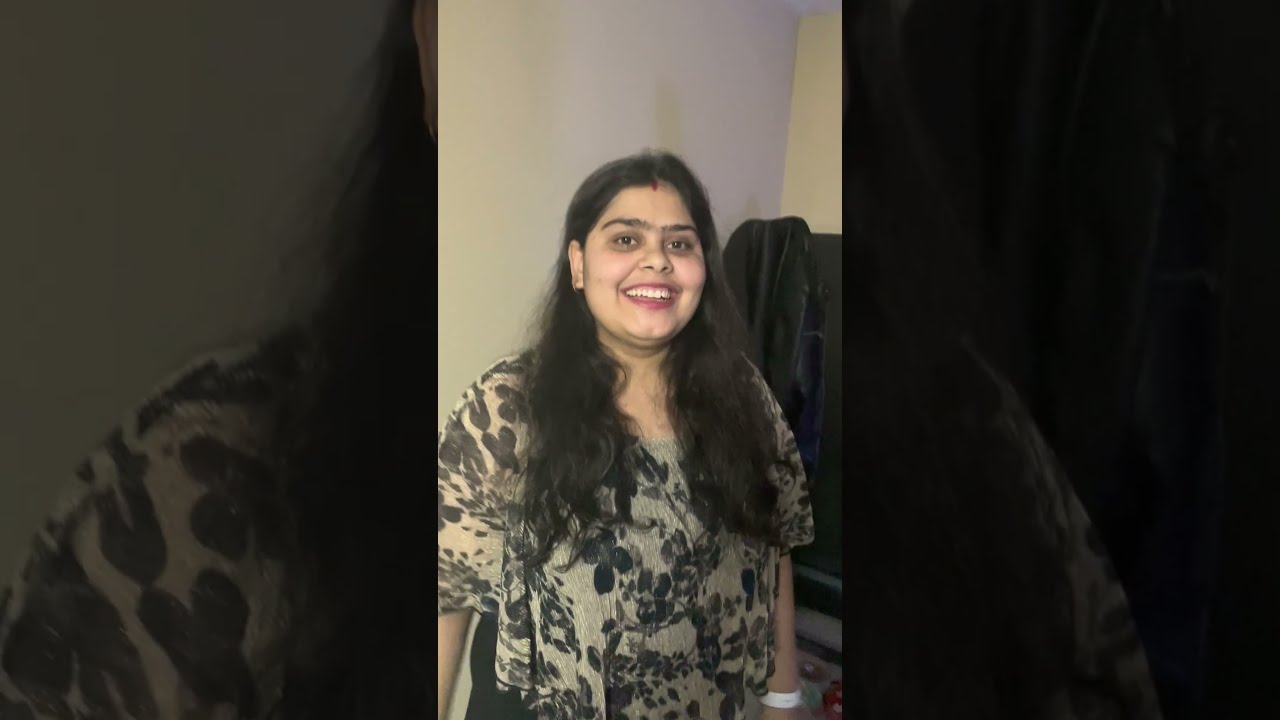In the center of the image stands a smiling woman with long, dark black hair, dark eyes, and pronounced dark eyebrows. She is dressed in a gray blouse adorned with black floral patterns and black pants. On her left wrist, she wears a white wristband. Directly behind her, where two walls meet, the left wall appears to have a light purple tint while the right wall is beige. A black jacket can be seen draped over a piece of black furniture in the background. Various colorful toys, predominantly purple, red, and green, are scattered on the floor. The image features thick borders on the left and right sides, which are created by enlarging and graying out elements of the main picture, adding depth and focus to the central scene.